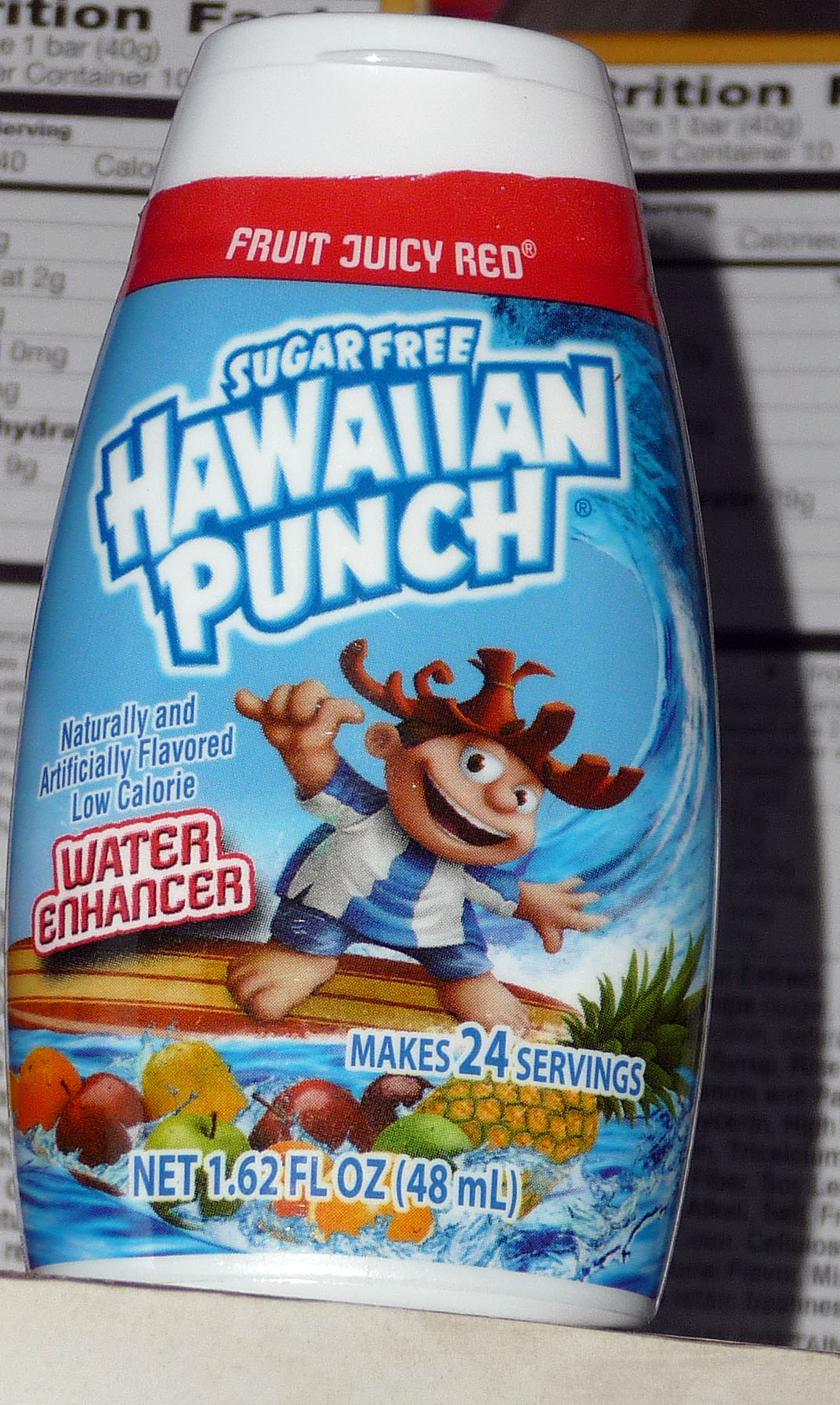This image features a small plastic container with a white lid. The container bears a prominent label that reads "Sugar-Free Hawaiian Punch" displayed in bold white letters, outlined in blue. Dominating the background of the label is an animated character of a child wearing a dark brown straw hat. The character is white, with a chunky face, hands, and feet, dressed in a blue and white striped shirt paired with blue shorts. The child is depicted riding a brown and tan striped surfboard on vibrant blue ocean waves, complete with white splashes. Interspersed among the waves are various fruits, including oranges, dark red apples, green apples, a pear, and a large pineapple positioned on the right side.

The label also includes additional text: "Naturally and Artificially Flavored, Low-Calorie Water Enhancer, Makes 24 Servings," followed by the net weight of "1.62 fluid ounces" or "48 milliliters." The container is resting on top of two other items that feature nutritional labels, providing additional context to the scene.